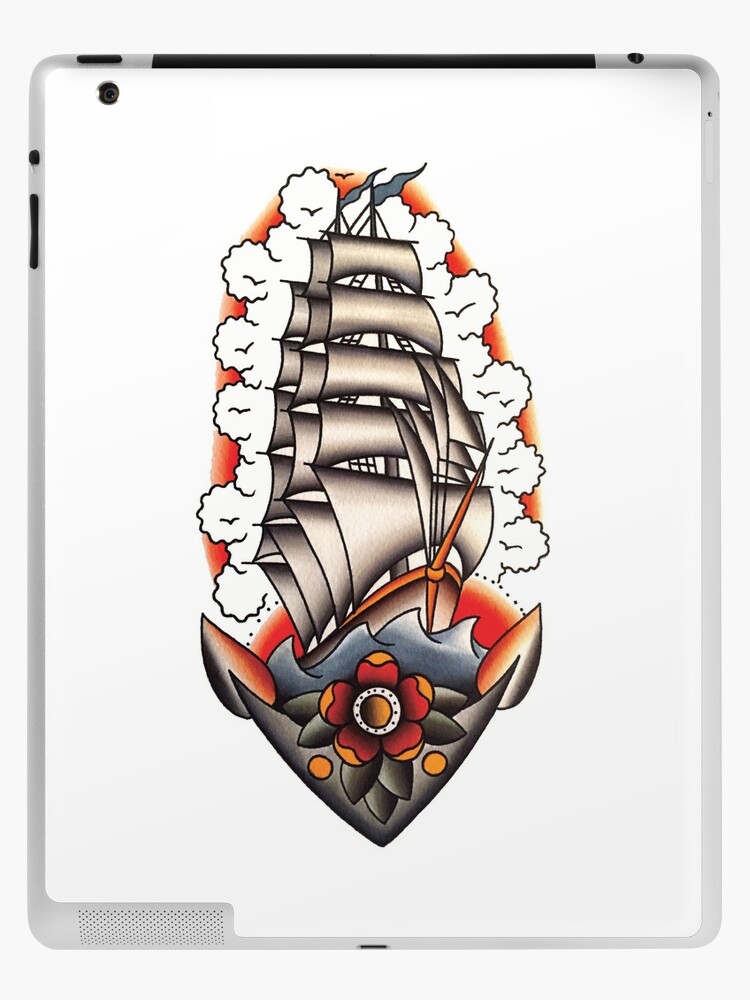This highly detailed illustration, set against a giant dry erase board with gray edges and black accents, portrays an elaborate pirate ship scene. At the base of the image sits a stylized gray anchor adorned with a vibrant flower, featuring gray leaves, orange and red petals, and an orange center. Above the anchor, stylized gray waves suggest a tumultuous sea.

The centerpiece of the illustration is a grand pirate ship. The hull is a mix of gray and brown hues, accented with orange details that add a touch of vibrancy. The ship's towering sails are an impressive blend of gray and white, rendered large and majestic against the backdrop. Behind the sails, the sky is filled with fluffy white clouds, each outlined in black for dramatic effect. Floating above, a few black seagulls add to the nautical atmosphere.

Further enhancing the scene, a hint of orange peeks out from behind the clouds, possibly indicating the glow of a setting or rising sun. Resting atop the ship are two grayish-blue flies, adding an unexpected and whimsical touch to this maritime tableau.